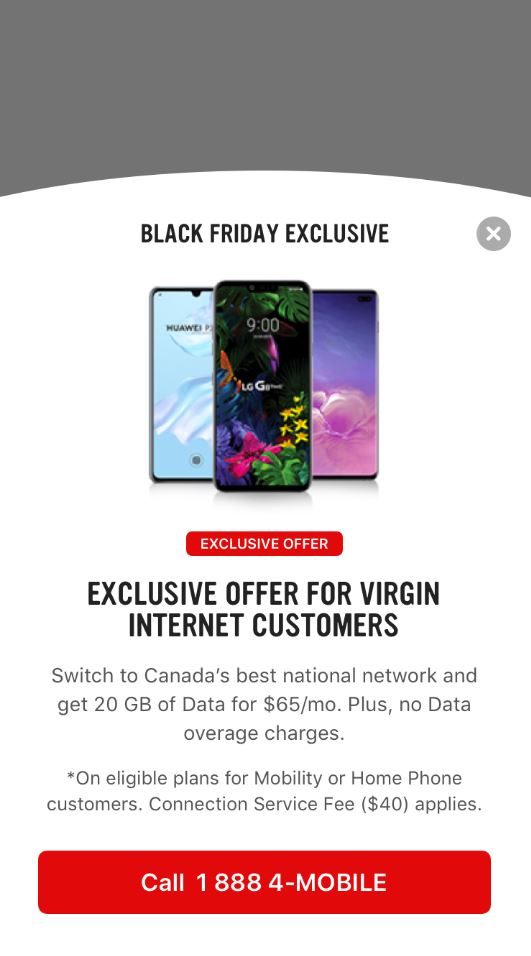This promotional image showcases a Black Friday exclusive offer from a website, designed with a sophisticated gradient that transitions from grey at the top with a rounded bottom edge into a white background. Dominating the center of the image is the bold, all-caps text "BLACK FRIDAY EXCLUSIVE" in a striking black font. To the top right corner, a small grey circle featuring a white "X" serves as a close button. Immediately beneath the headline, three cell phones are prominently displayed, with one phone in the foreground and two slightly behind it, emphasizing the tech-related nature of the deal.

Further below, there is a button-like banner labeled "EXCLUSIVE OFFER," drawing attention to the call-to-action. Under this banner, the text "EXCLUSIVE OFFER FOR VIRGIN INTERNET CUSTOMERS" is clearly stated, targeting a specific customer base. The final section of text unveils the specifics of the promotion: "SWITCH TO CANADA'S BEST NATIONAL NETWORK AND GET 20GB OF DATA FOR $65 A MONTH PLUS NO DATA OVERAGE CHARGES," highlighting the deal's compelling features and benefits.